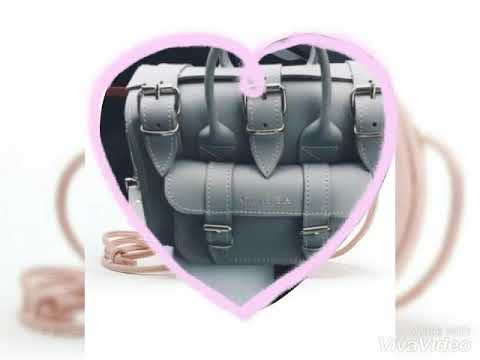The image is a grayscale photo of a dark black leather purse with three straps across its top – one strap on each side and one in the middle, situated between the purse handles. Below the main compartment, there's an additional pocket that features two more straps. The entire purse is framed within a pink, hand-drawn heart outline. The background of the image is predominantly white with what seem to be small rubber bands at the bottom. In the bottom right corner, a slightly pixelated and faded watermark reading "Viva Video" can be seen. Due to the background and heart outline, the focus is on the luxury aspects of the purse, highlighting its numerous compartments and intricate design.